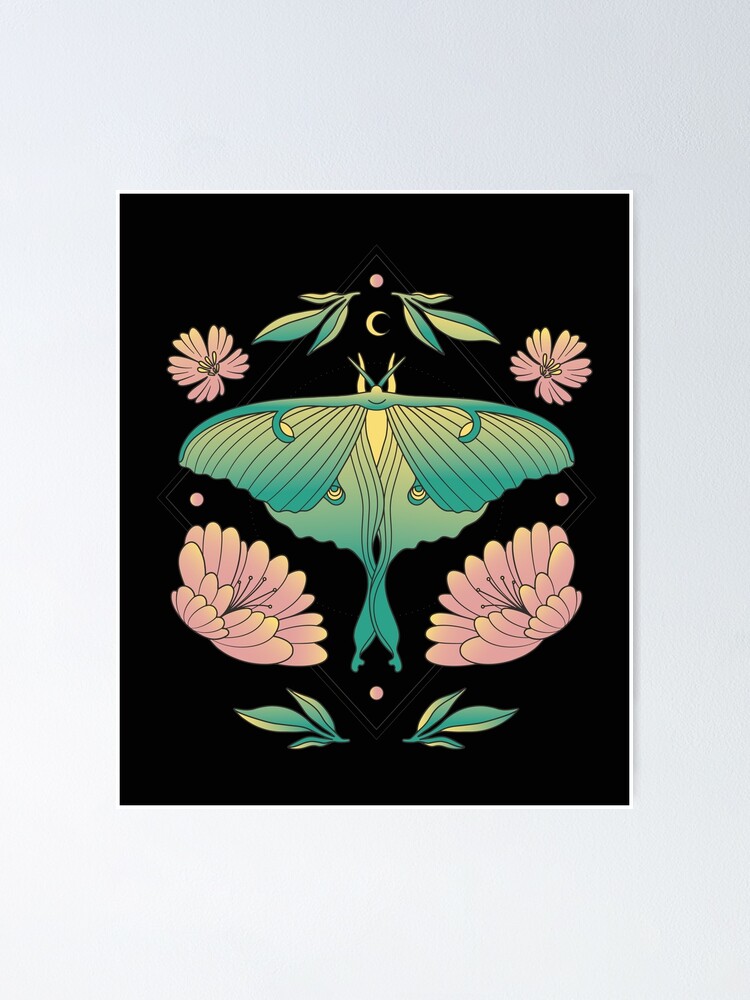This is a detailed digital illustration framed in white against a white wall. The artwork features a central, turquoise-green butterfly with a black background, resembling black paper, emphasizing its vibrant coloration. The butterfly, which has discernible eyes and a mouth, is the focal point, appearing to gaze directly at the viewer with its yellowish eyes. Above the butterfly hovers a crescent moon, flanked by dots, and surrounded by a diamond-shaped arrangement. Encircling the butterfly are four pink flowers, two smaller ones on either side of the moon and two larger ones below, resembling daisies. Complementing this arrangement are two sets of leaves: one set at the top and one set at the bottom, each with leaves extending left and right. Adding to the symmetry and color balance, pink dots are positioned at each corner of the artwork, creating a cohesive and enchanting composition.